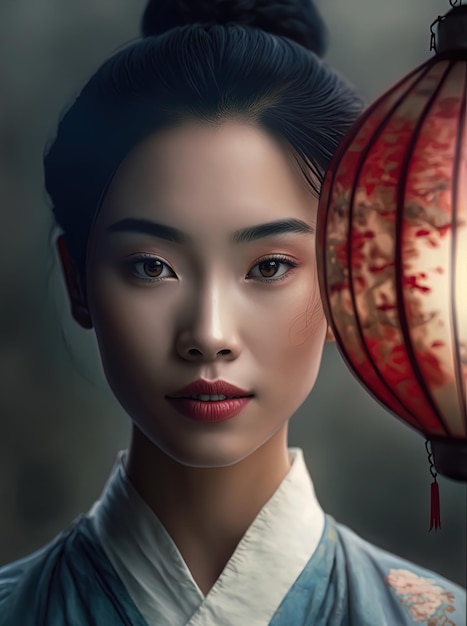This is a detailed portrait of a young, beautiful Asian woman, likely Chinese or Japanese, who is standing and facing the camera. The image captures her from the neck up, with her black hair elegantly styled in a bun behind her head. She is wearing a blue kimono or dress that has a white collar forming a V-shape at her neck, and there's a painted floral design on her right shoulder. The woman's expression is somewhat stoic, accentuated by her arched eyebrows and red lipstick, giving her a very composed and focused look.

In the foreground, to the right of the woman, is a lit lantern with red polka dots and black lines running down its spherical shape. The lantern's light adds a warm glow to the scene, contrasting with the gray background. Only half of the lantern is visible within the frame, positioned at the edge of the image. The woman’s brown eyes and well-kept eyelashes further enhance her refined appearance. The overall composition of the image is minimalist yet striking, highlighting both the woman's delicate features and the intricate details of her attire and the lantern. This sophisticated and visually appealing image might be AI-generated.